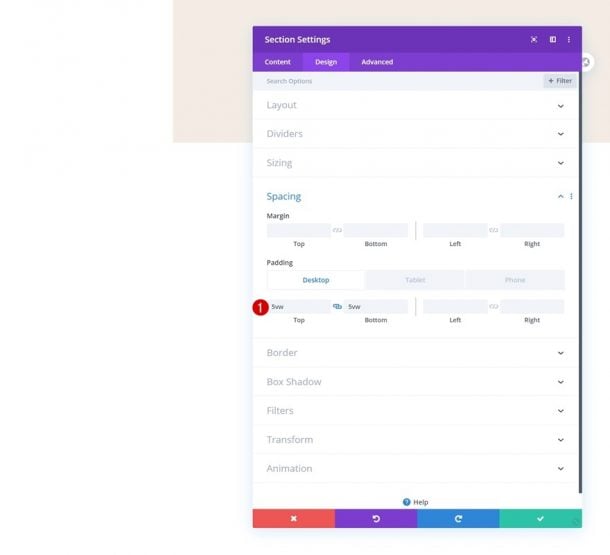This image is a cropped screenshot showcasing a segmented settings panel set against a colorful background. The settings panel itself is predominantly purple and overlays a multicolored page. At the top of the panel, there is a sizeable, light pink rectangular section, under which the background shifts to white.

On the far right at the top of the panel, there are three icons arranged from left to right: a maximize icon, a page view icon, and a menu icon. Below these icons, the panel is divided into three main categories: Content, Designs, and Advanced, with the Designs category being selected.

Directly below this header, the background turns white again with the title "Search Options" displayed at the top. To the far right, a filter button is prominently featured. Under the "Search Options" title, the options listed are "Layout," "Dividers," and "Sizing," each accompanied by a drop-down arrow for further customization. 

The "Spacing" option follows these categories and is highlighted in blue. An up-pointing arrow indicates that the spacing settings are currently expanded. Within the spacing section, there are settings for "Margin" and "Padding," alongside a box labeled "SVW." The SVW box has a red circle with the number one to its left. Below this, there are options for "Top" and "Bottom" spacing, linked by a chain icon in the center of the boxes aligned with the number one.

Further down the panel, more drop-down options are listed: "Border," "Box Shadow," "Filters," "Transform," and "Animation." At the very bottom, centered in tiny gray text, the word "Help" appears. Next to "Help," a small blue circle contains a question mark, indicating a help feature or guide.